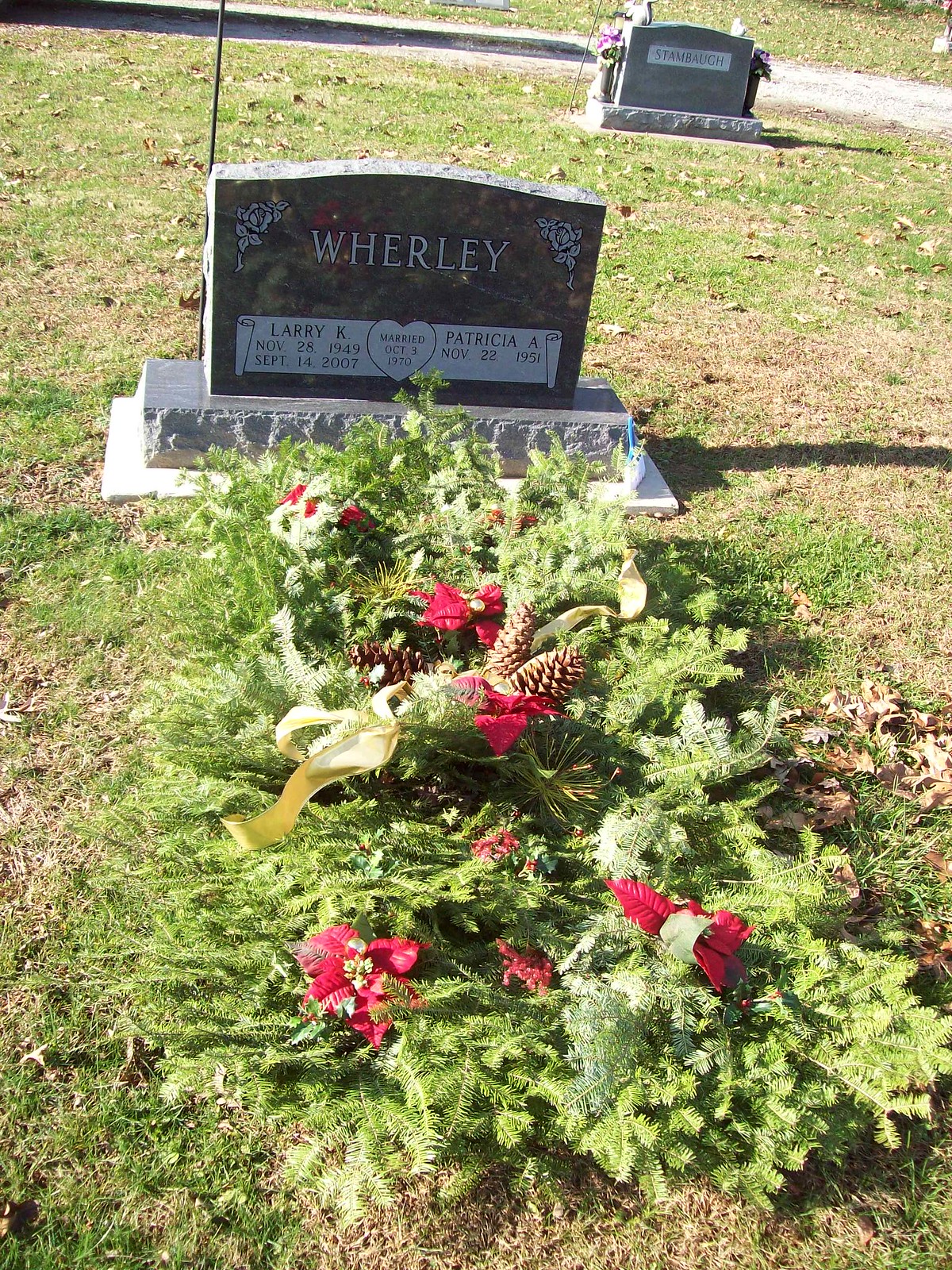This is a photograph taken inside a graveyard, showcasing a small gravestone in the foreground. The gravestone bears the name "WORLEY," spelled W-H-E-R-L-E-Y, inscribed in capital letters near the top. At the very bottom of the image, white text appears on a white background. The gravestone is situated on a grassy patch, which varies in color from light yellow to light green, indicating it might be the non-growing season when grass starts to brown out.

In front of the gravestone lies a large, elaborate arrangement of greenery, resembling a splayed-out wreath or a collection of wreaths. This festive display includes pinecones, red ribbons, yellow ribbons, and elements of pine, suggesting a holiday theme. The arrangement, with its Christmas-y look, includes red poinsettias and is likely placed there to commemorate the season.

In the background, another small gravestone can be seen with a few flowers placed to its left. Further beyond, there is a path and additional grassy areas. The ground around the gravestones is adorned with cut grass, leaves, and twigs, further emphasizing the wintery context of the scene.